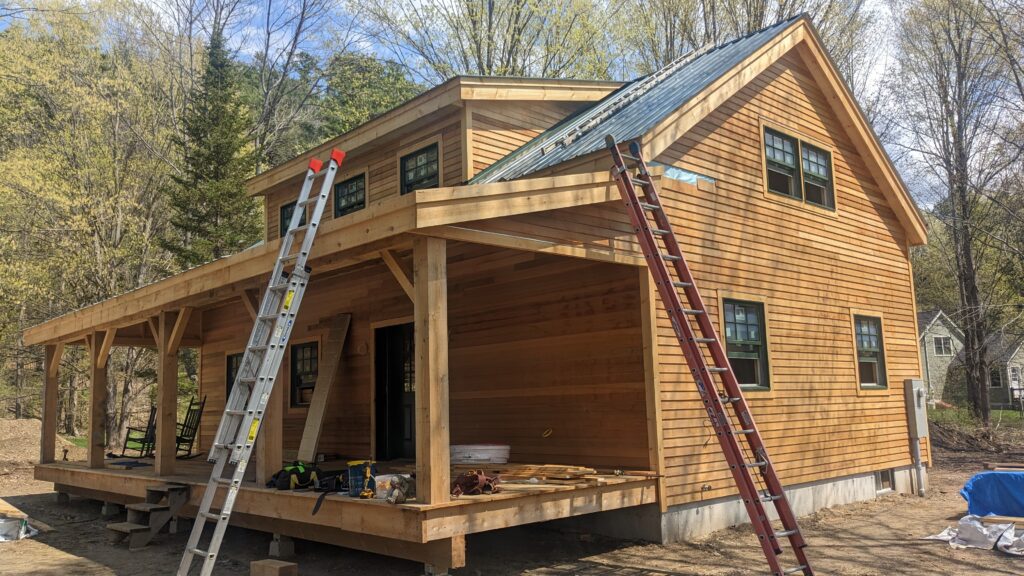The image depicts a two-story house under construction in a wooded area with a clear blue sky and some low-lying clouds. The house, resembling a charming cottage or cabin, is primarily constructed from cedar wood and features a metal roof that is being installed. The expansive front porch, which spans the entire length of the house, hosts two rocking chairs and a set of three wooden steps leading up to it. Tools and a gray basin are also visible on the porch. You can see a red ladder leaning against the side and an aluminum ladder at the front, reaching up to the roof. The ground around the house is bare dirt, indicating ongoing development. The house has numerous windows, including four on the front facade—two on the ground floor and two connected at the top. There's also an open door frame and visible structural beams. Big trees, including pine trees, surround the construction site, and another home can be seen in the background.